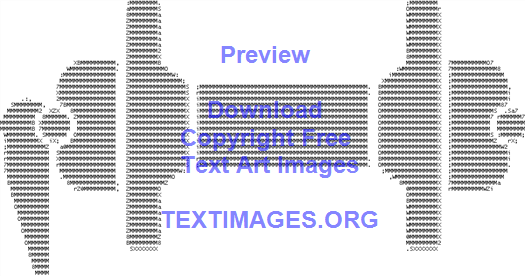The image displays a low-resolution, grayscale, computer-generated graphic on a white background. The graphic appears to be an abstract or indiscernible object, possibly resembling a dumbbell, bicycle with a kickstand, or a screw with a handle and knobs, composed of black and gray characters and lines. Overlaid on the image is text in purple, reading "Preview," "Download," "Copyright Free," and "Text or Images." Additionally, the bottom of the image features the website, "TEXTIMAGES.ORG," also in purple. The overall quality of the image suggests it is a piece of clip art, intended to be copyright-free.